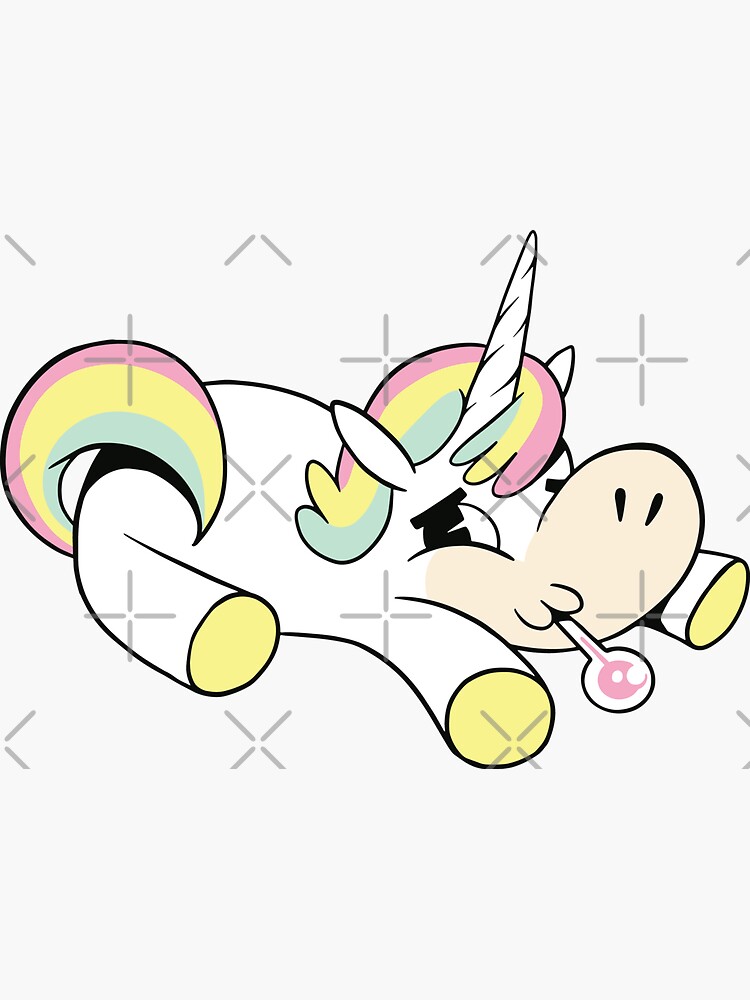This detailed illustration depicts a charming baby unicorn, lying on its belly with its legs adorably stretched out. The unicorn, with its pristine white body and large, pronounced white horn emerging from its forehead between its ears, faces right at a three-quarter angle. It boasts a vibrant rainbow mane and tail, featuring hues of pink, yellow, and baby blue. Its tail curls upward over its back. The unicorn's large, expressive oval eyes with black pupils add to its endearing appearance. Despite a minor confusion, it holds a baby's pacifier – initially mistaken for a thermometer – in its mouth, adding a further touch of innocence. The scene is set against a pure white background, adorned with gray cross and check mark watermarks, which serve to protect the artwork from unauthorized use.